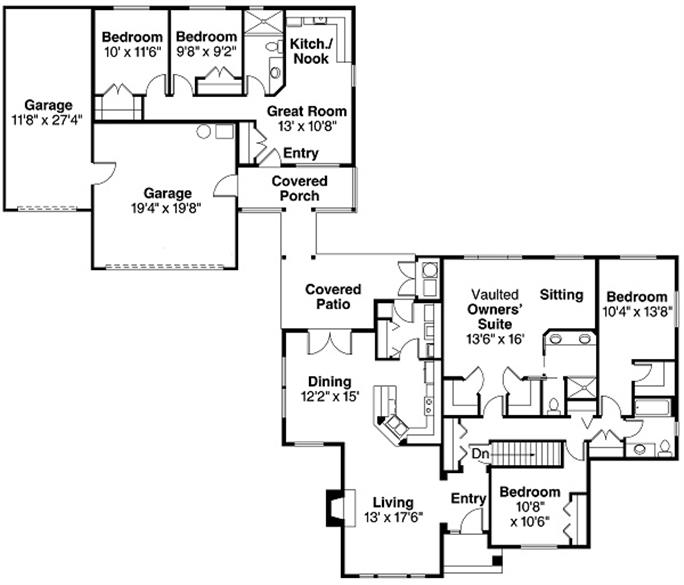The diagram illustrates two interconnected floor plans of houses, joined by a small path extending to their covered patios. The upper left floor plan features a garage on the far left, followed by two adjacent bedrooms. Below these bedrooms is a larger, square-shaped garage. On the right side of the plan, there's a kitchen nook at the top, a great room below it, and an entrance leading to a covered porch at the bottom. The lower right floor plan includes a covered patio at the top left corner, with a dining room situated below. To the right of the dining room is the vaulted owner's suite, and adjacent to it on the far right is another bedroom. Below the suite is an additional bedroom, with a living room and an entry placed to the left. These two distinct sections are connected through the covered patios, forming a unique, cohesive architectural layout.